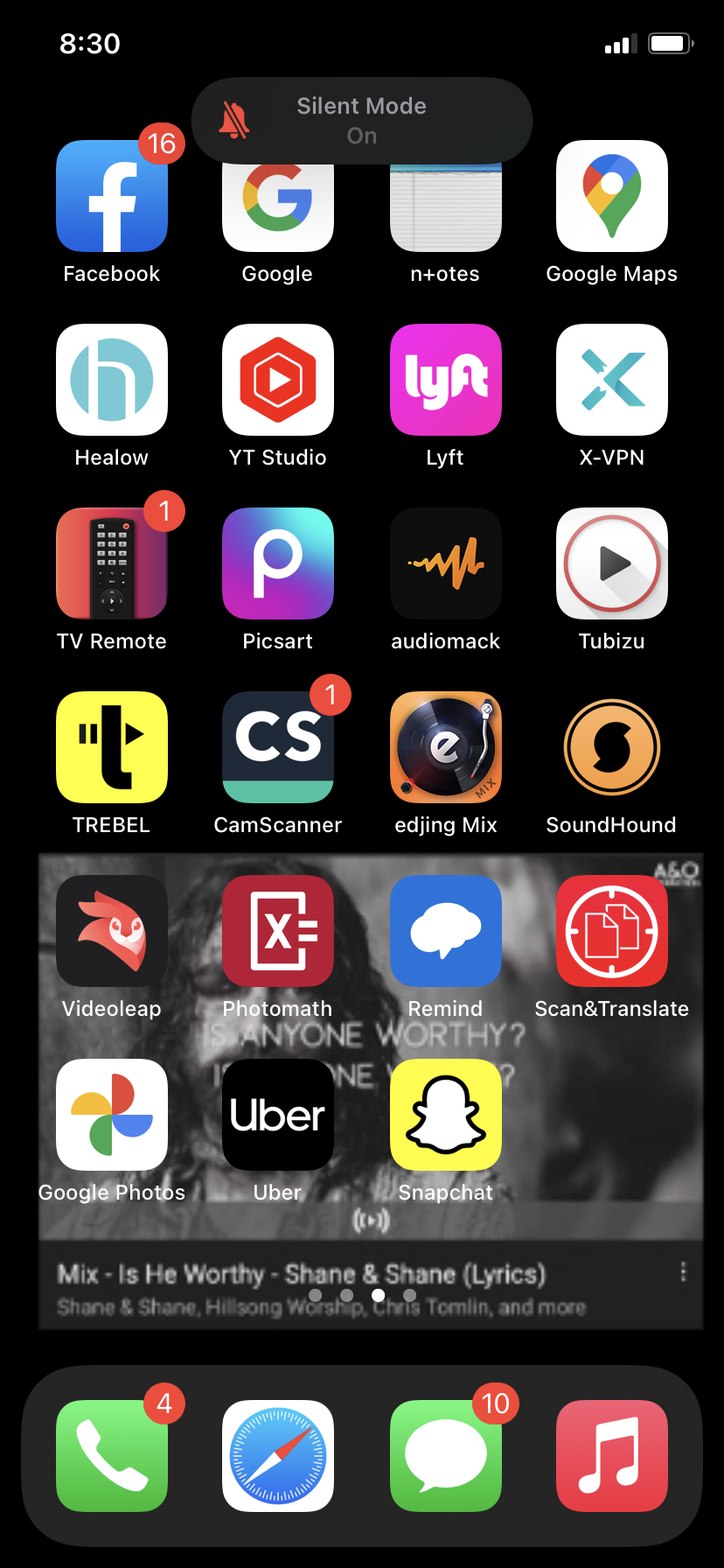The image displays the home screen of an iPhone. Along the bottom of the screen, there's a green Phone icon, indicating the user has four missed calls or voicemails, as shown by a red notification badge. Next to it, the Safari icon is prominently visible in white and blue colors. The Messages icon is green with a white speech bubble in the center and has a red notification badge indicating ten unread messages. The Music icon is also visible with a red and white design. 

The home screen is populated with various app icons including Facebook, Google, Google Maps, Lyft, TV, Remote, and The Hill. In addition, in a gray-colored section towards the middle of the screen, icons for Snapchat, Uber, a Scan and Translate app, and the Remind app are present. Some icons are difficult to identify due to their small size.